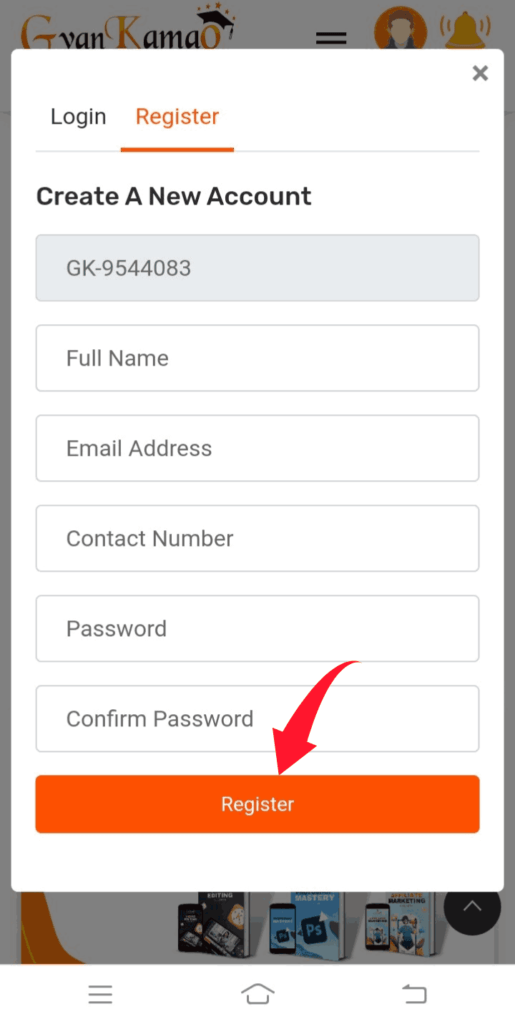This image is a detailed screenshot taken from a mobile device, showcasing a registration page on a website named "PINMOA". The distinctive branding of the site includes the name "PINMOA" with the final 'O' adorned with an academic graduation cap. The background features a variety of educational resources, including books, audiobooks—illustrated with an image of a book next to a phone. At the top of the page, there are account management options such as profile, notifications, and possibly settings.

The main focus of the screenshot is the registration form, which offers two options: 'Login' and 'Register,' with the 'Register' option currently selected. The form begins with a section labeled "Create an Account" and consists of multiple fields for user information. The first field appears to be auto-filled with "GK9544083," likely the device ID of the phone used to capture the screenshot. Subsequent fields require the user’s full name, email address, contact number, password, and confirmation of the password. At the bottom of the form is an orange "Register" button. 

A prominent red arrow is superimposed on the image, pointing towards the registration form, indicating that this screenshot likely serves instructional or guided purposes to help users understand how to fill out the registration details.